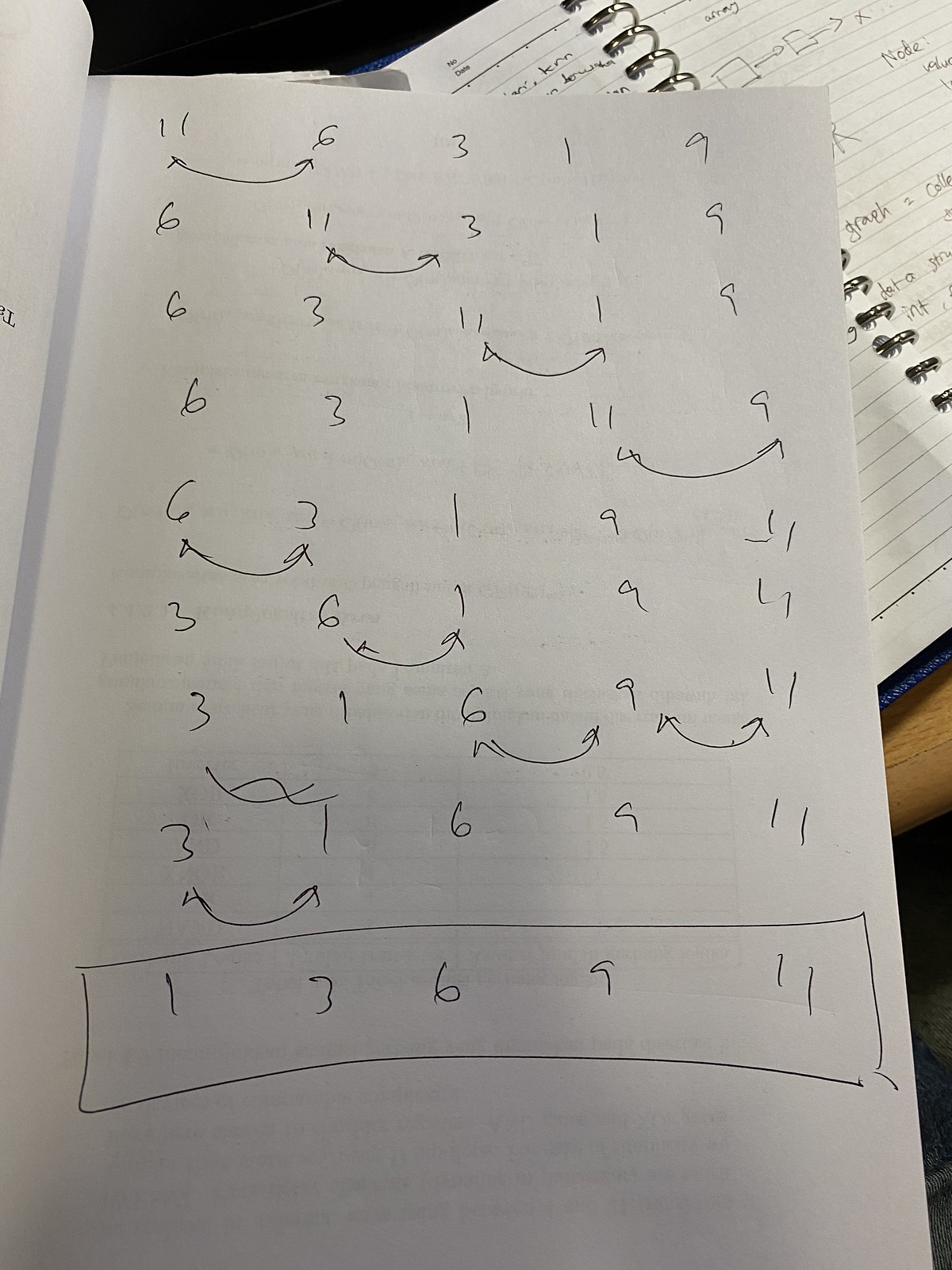The photograph is a vertically oriented color image featuring a sketchbook that occupies most of the frame, except for a small portion in the top right corner where the background is visible. The sketchbook is open to a white sheet of paper covered in pen marks. At the bottom of the page, there is an outlined box that contains the numbers 1, 3, 6, 9, and 11 written in succession. The upper portion of the page is dotted with numbers linked by arrows, seemingly indicating some flow or sequence, possibly forming a flowchart or diagram that illustrates a process involving these numbers.

Beneath the white sheet of paper lies a hardcover spiral-lined notebook, partially visible. This notebook also has black pen marks, including text and symbols such as a square, an arrow, and an 'X' that suggest mathematical or engineering notations. The diagrams and markings on the white paper and the open notebook allude to a detailed and intricate planning or computational process.